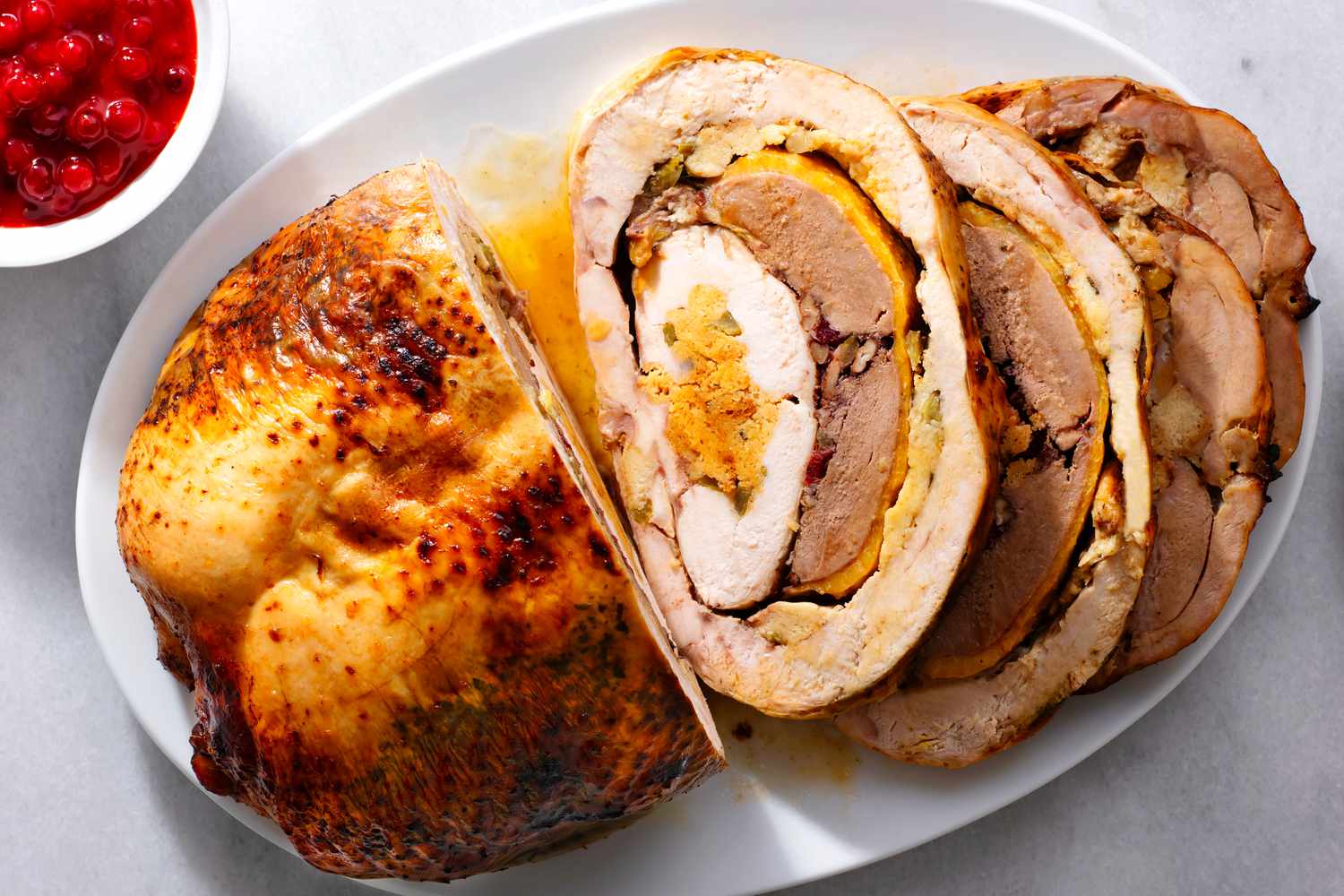The image showcases a beautifully prepared and plated meat dish, viewed from above. The centerpiece is a stuffed and rolled roast, displayed on an oval white china platter. The roast is artfully sliced into four pieces, revealing intricate layers. The outermost layer is golden-brown and crispy, likely turkey or chicken skin, indicating a well-roasted finish. Inside, there's an array of fillings: a darker meat layer, a white meat layer, and what looks like a hard-boiled egg encased within. Additionally, there is a vibrant orangey-yellow layer, which could be cheese or a type of stuffing, adding to the dish's visual and culinary complexity. Nestled beside the main portion on the platter, the layered slices lie atop a bed of bright yellow meat juices, further enhancing the roast's appeal. In the upper left-hand corner of the image, there is a partial view of a white ceramic bowl containing what appears to be jellied cranberries or cranberry sauce, suggesting a festive or holiday meal setting. The entire presentation rests on a white marble-like surface, adding a touch of elegance to the culinary display.